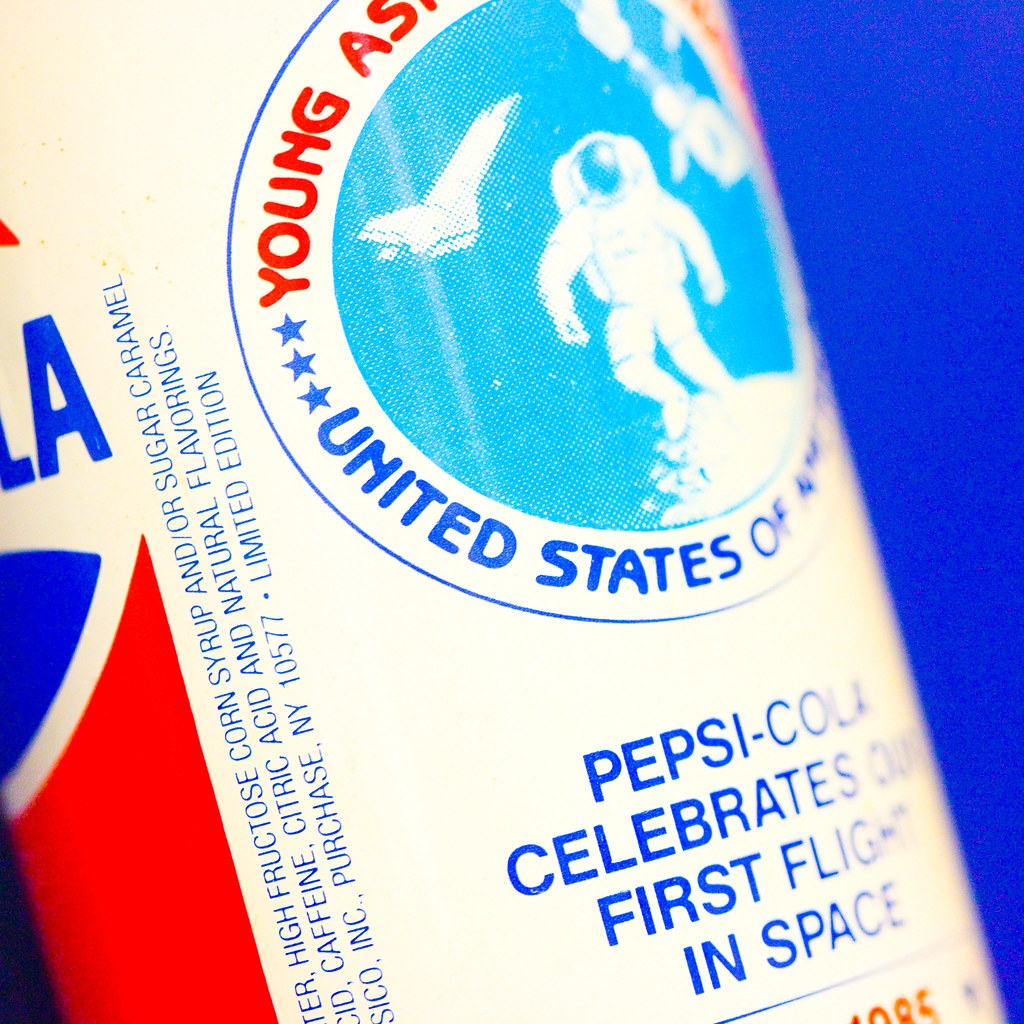The image is a color photograph in a square format, showcasing a close-up of a white Pepsi-Cola can. The can is angled from the top left to the bottom right, with a prominent commemorative logo situated midway. This logo is circular, featuring a light blue background with a white outline of an astronaut and a jet overhead. The perimeter of the circle contains red typography that partially reads “Young Astronaut,” and blue text with three stars saying “United States of," with the rest cut off. Below this, additional blue text states, “Pepsi-Cola celebrates first flight in space.”

The left-hand side of the can displays ingredients in blue writing, including high fructose corn syrup (and/or sugar), caramel, caffeine, citric acid, and natural flavorings. The can also mentions "Purchase NY10577 limited edition." The top section of the can features segments of red, white, and blue, with partial letters that appear to spell "LA." The date "1985" is visible at the bottom of the photograph, giving it a vintage feel.